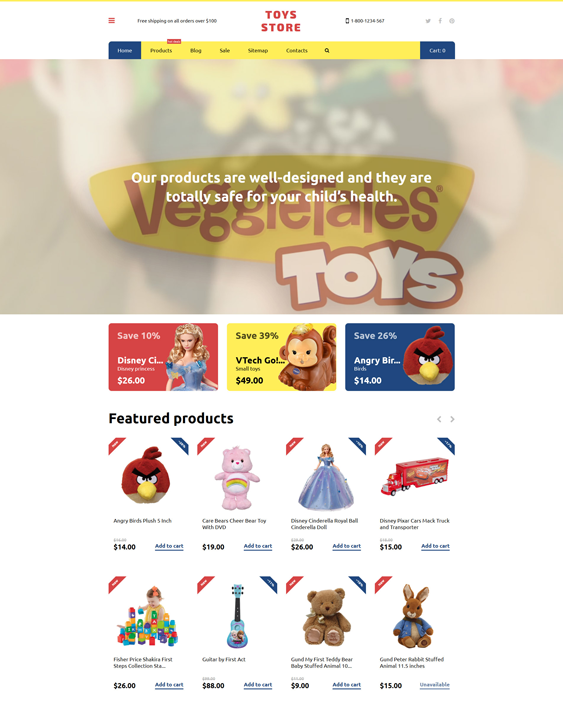This image is a screenshot of the homepage of a website called Toy Store, easily identifiable by the bright red "Toy Store" logo prominently displayed at the center top of the page. Just below the title, a menu bar is visible, featuring categories with blue backgrounds on the edges and yellow backgrounds for the categories in between.

The main section of the homepage features a large banner image. The background of the banner is yellow with the text "VeggieTales" written in red font and the word "toys," in large, bold white font with a red outline, positioned slightly to the right below "VeggieTales." Superimposed on this image is promotional text in white font that reads, "Our products are well designed and they are totally safe for your child's health."

Below the VeggieTales banner are three promotional images. On the bottom left, there is an image of a female princess doll with blonde hair and a blue dress, against a red background. White text to the left of the doll reads, "Save 10%," followed by "Disney," and "$26." The center image features a monkey doll on a yellow background, with black text to the left that reads, "Save 39%," "VTEC," and "$49." The image on the right shows an Angry Bird plush on a blue background, with white text on the left reading, "Save 26%," "Angry Birds," and "$14."

Further down, two rows of featured products are displayed. The top row from left to right includes:
1. Angry Bird plush for $14
2. Care Bear for $19
3. Princess doll for $26
4. Toy truck for $15

The row below shows:
1. Cup stacking game for $26
2. Toy guitar for $48
3. Teddy bear for $9
4. Rabbit plush wearing a blue jacket for $15

Each featured product has its price in the bottom left corner and an "Add to Cart" button in the bottom right corner, allowing for easy shopping.